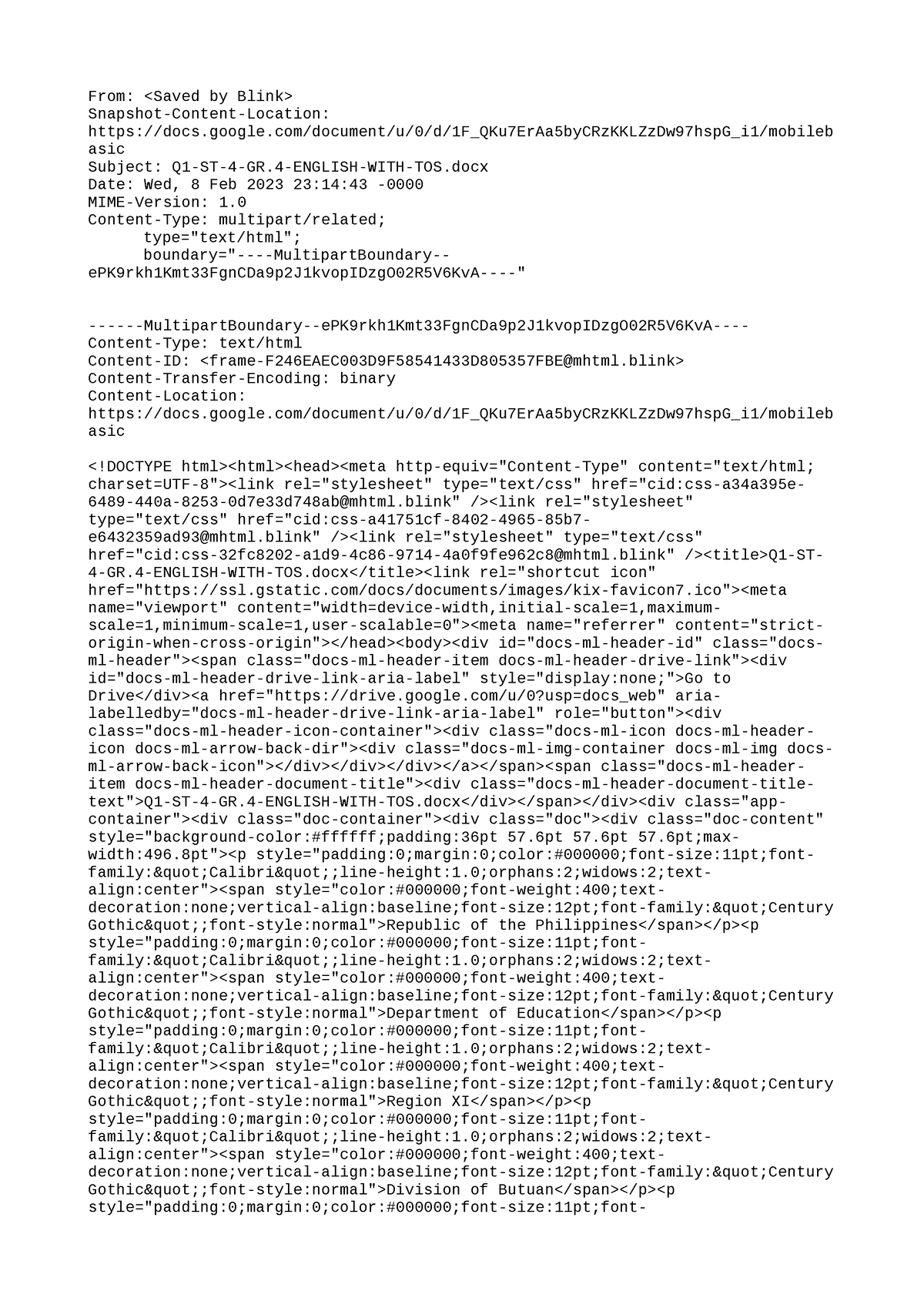An image displaying a dense block of black text on a white background. The text includes a URL: https://docs.google.com/document, followed by a series of metadata details. These details encompass information such as subject, document type, version, content type, and character encoding. The description mentions the subject "Q1-ST-4-Gr. for English with TOS," a date and timestamp "Wednesday 8 February 2023 23:14:43," and various HTML-related tags and attributes. The layout is in an HTML format, indicating an email or document metadata, with references to multi-part boundaries and encoding methods.